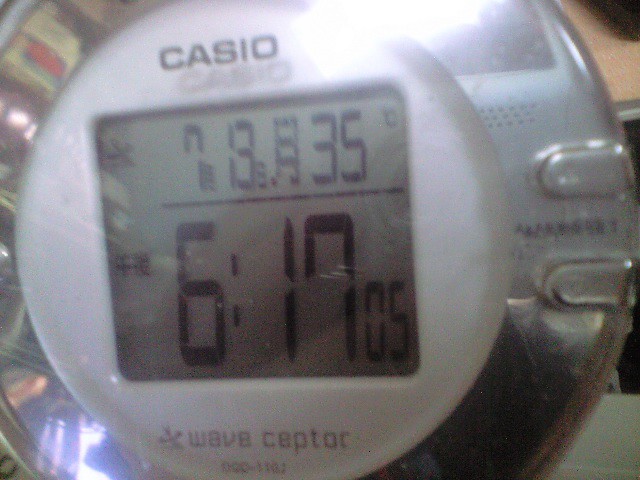This image showcases a close-up view of a stopwatch. The stopwatch features a round shape with a prominent stainless steel border and a white face panel. Within this panel lies a square digital screen displaying the numbers "7:13:35" with a line beneath this value. Below this line, another set of numbers reads "6:17:05."

At the top of the digital screen, the brand "CASIO" is prominently displayed in bold, uppercase black letters. Below the screen, the label "Wave Ceptor" is inscribed in silver. The stopwatch is protected by a glass covering.

The image also reveals the presence of two oval-shaped buttons situated on the right side of the stainless steel border. Due to the close-up nature of this photograph, only a portion of the stopwatch is visible.